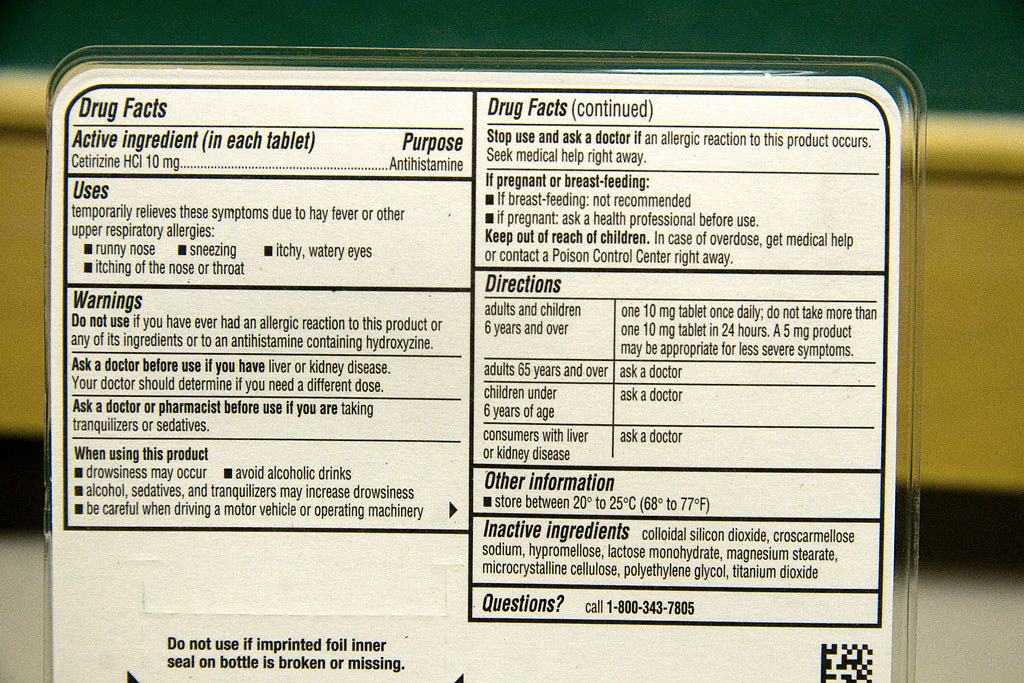The image depicts a high-quality close-up of the drug facts label on the back of a plastic, vacuum-sealed medicine package, specifically for cetirizine HCL 10 milligram tablets. The photo reveals detailed information about the medication, including its use as an antihistamine for temporarily relieving allergy symptoms such as runny nose, sneezing, itchy and watery eyes, and itching of the nose or throat. The background shows a blurry classroom setting with a chalkboard, indicating the photo was likely taken in an educational environment but emphasizes the medication as the primary subject.

The active ingredient listed is cetirizine HCL 10 milligrams. The label provides clear warnings, such as avoiding use if there's a history of allergic reactions to this product or any antihistamines containing hydroxyzine, and advises consulting a doctor if you have liver or kidney disease. It emphasizes that users should avoid alcoholic drinks and be cautious when driving or operating machinery due to possible drowsiness. Dosage instructions specify that adults and children aged six and over should take one 10 milligram tablet daily, not exceeding one tablet in 24 hours. Special instructions are given for adults over 65 and children under six, advising them to ask a doctor before use. The product should be stored between 20 and 25 degrees Celsius (68 to 77 degrees Fahrenheit).